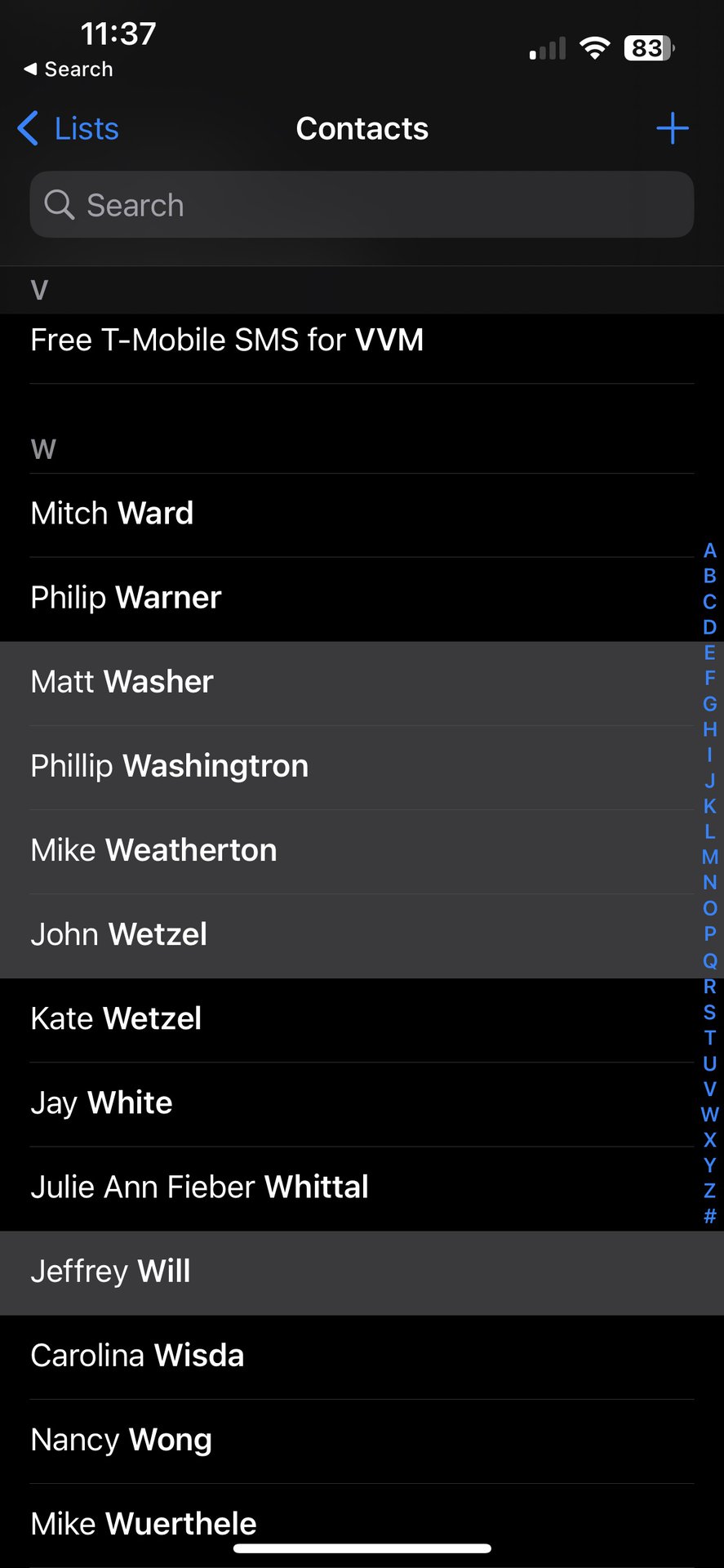The image shows a phone screen displaying several user interface elements. At the top, the screen shows a Wi-Fi signal icon with one bar and the number "83" next to it, indicating signal strength or battery percentage. The time displayed is "11:37." Below this, in small print, is the word "search" with an arrow pointing left. Further down, a blue arrow labeled "Lists" points left, accompanied by a white "Contacts" label and a blue cross on the right side, suggesting clickable or interactive elements.

Beneath this, a lighter, shaded rectangular box contains the word "Search" along with a magnifying glass icon, indicating a search function. The content below lists several contacts, with some names in grayscale: "Free T-Mobile Sims for VVM," "Mitch Ward," "Philip Warner," "Matt Washer," "Philip Washgank-Trunn," "Mike Weatherton," "John Wetzel," "Kate Wetzel," "Jay White," "Julie Ann Fiber-Whittle," "Jeffrey Will," and more. Notably, several contacts—"Matt Washer," "Philip Washington," "Mike Weatherton," "John Wetzel," "Jeffrey Will," and possibly others—are grayed out, differentiating them from the others, which could indicate inactive or unavailable contacts. Additional names include "Carolina Wisda," "Nancy Wong," and "Mike Werthel."